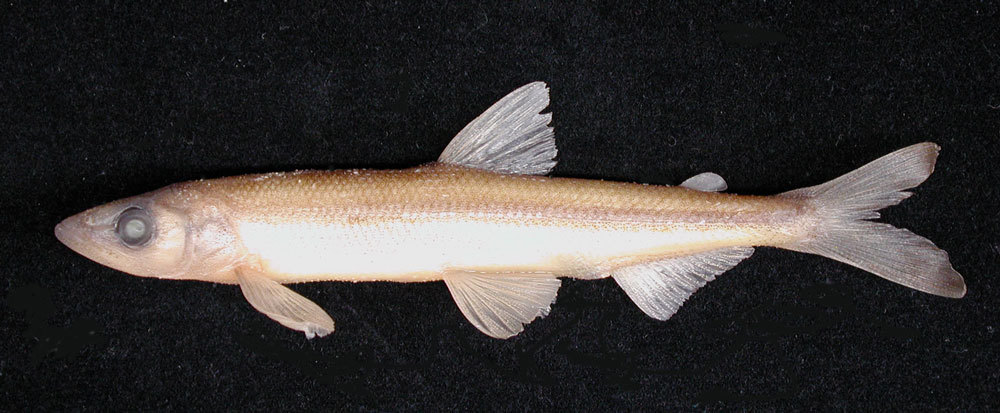This is an image of a small, long, and very thin fish, possibly laid out for scientific research, set against a black background with tiny white specks resembling a black piece of velvet. The fish appears to be dead, and its body displays a gradient from a translucent, light brown color on top to a bright white belly. The fish has a side-facing composition with a visible grayish, cloudy eye, giving it a slightly eerie, deep-sea appearance. The creature's thin fins are also translucent and delicate, with a detailed arrangement: a large tail fin flows to the left, followed by a smaller fin on the top and a larger one at the bottom. The middle part of its body features two more fins—one on top and another on the bottom—while a final smaller fin is located closer to the head on the underside. The fish is illuminated by a bright light that accentuates the stark difference in coloration between its top and bottom.